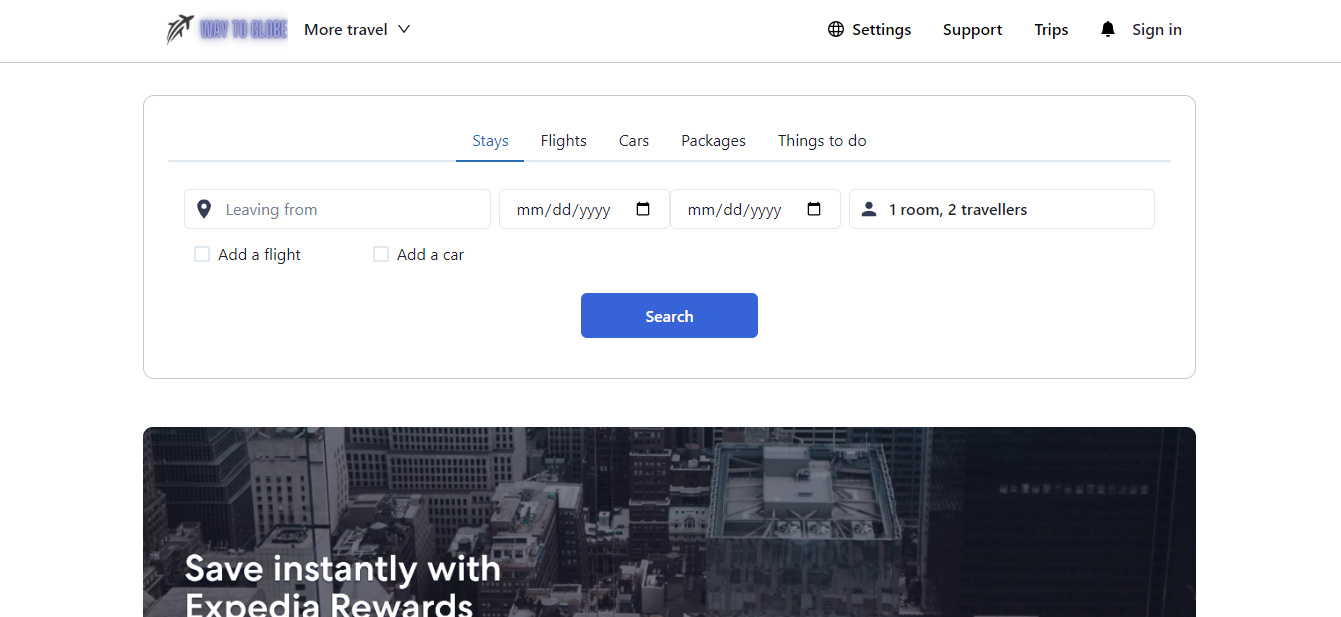This image captures a sleek and organized travel booking homepage. At the top, a user-friendly menu offers easy navigation with options including Settings, Support, Trips, and Sign In, along with additional travel resources. Below this, users can begin their search within clearly defined categories such as Stays, Flights, Cars, Packages, and Things to Do. The search functionality allows users to input departure cities, travel dates, room preferences, and the number of travelers. Additional options are available to include a flight or car rental. A prominent search button sits just below these input fields, ready to initiate the booking process. Dominating the visual space of this screenshot is a stock aerial view of a city, accompanied by a banner text promoting savings with Expedia Rewards. The remaining components of the homepage, not visible in this cropped screenshot, maintain a clean and minimalist aesthetic with a mostly white background, ensuring an uncluttered and efficient user experience.